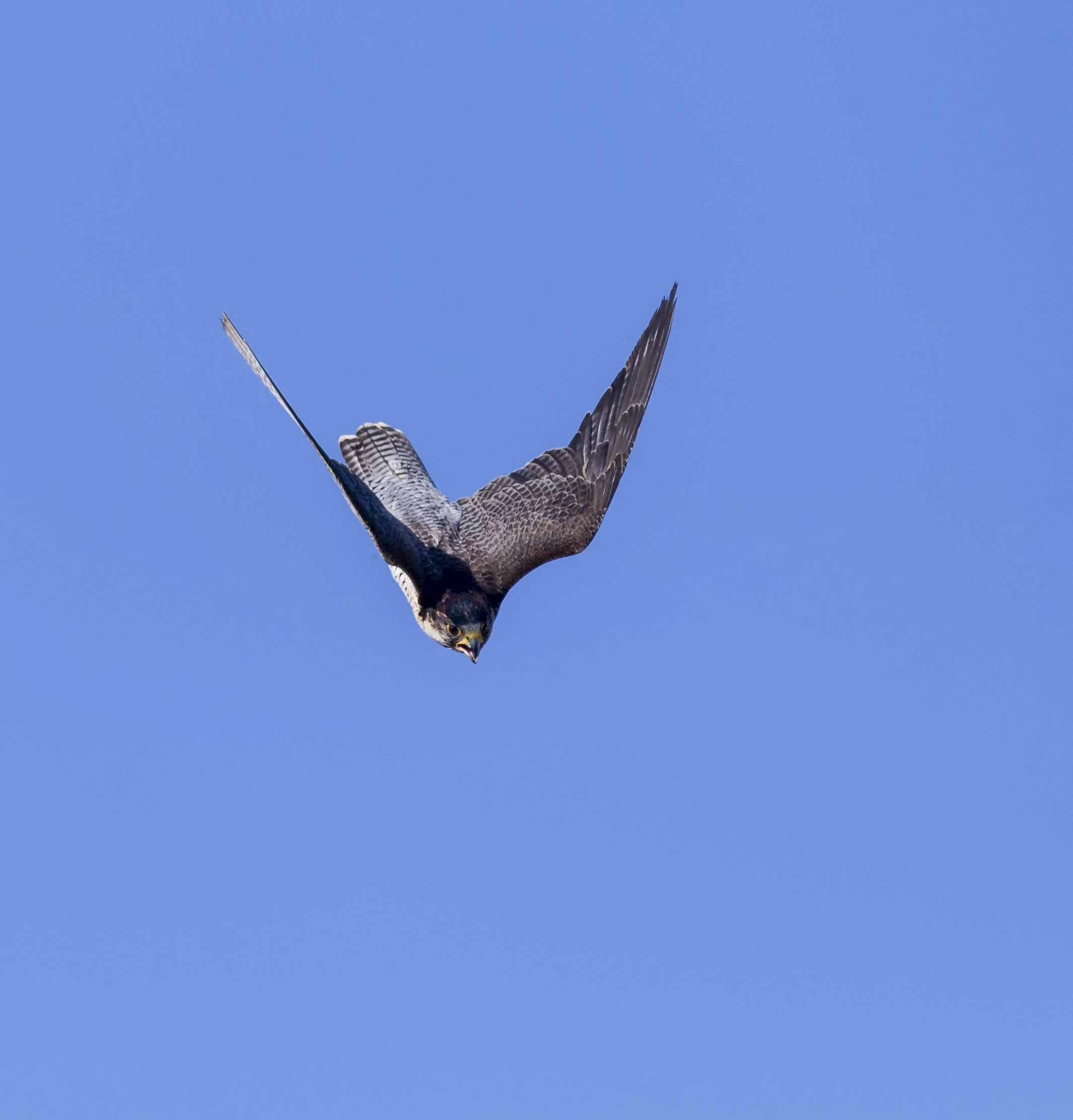The image captures a majestic aerial scene set against a clear, medium periwinkle blue sky with subtle blends of purple hues. At the center of this tranquil yet dynamic sky, a formidable bird of prey, possibly a hawk or a falcon, executes a breathtaking dive towards its unseen target below. The bird's powerful wings are outstretched and angled upward, showcasing their impressive span and pointed tips. Its plumage is a striking combination of gray, black, and white, with darker tones on its back and hints of white on its breast and throat. The bird's sharp yellow beak is slightly open, revealing a pink tongue, adding to the intensity of the moment. Its focused, round black eyes pierce the scene, emphasizing its concentration and predatory intent. The bird's sleek, elongated tail extends behind it, mirroring its streamlined dive. A slight shadow plays across its back, accentuating its three-dimensional form against the sky. This dramatic and vivid depiction resembles a moment worthy of National Geographic, capturing the raw elegance and precision of a bird of prey in action.